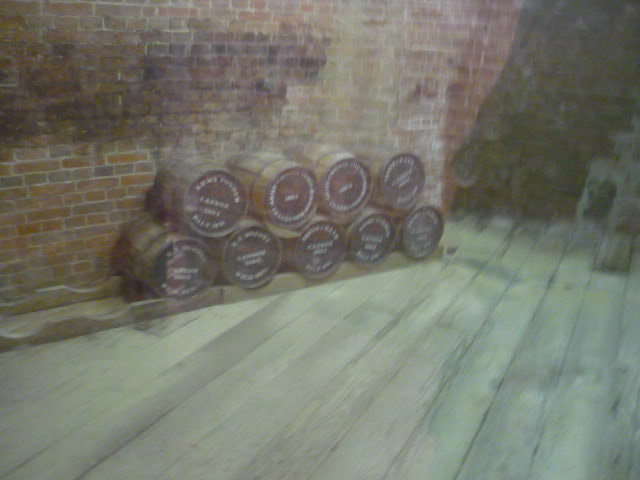In this low-resolution and somewhat blurry photograph, we are presented with a cozy, rustic scene that appears to be inside a cellar of a brick building. The floor is comprised of white or pale grey wooden slats reminiscent of flooring in an old tavern from a western movie. Dominating the image are nine dark wooden kegs, arranged in a staggered formation with five kegs on the bottom row and four kegs nestled in the gaps of the five beneath them. Each keg rests securely on a timber rail designed to fit their curved shapes.

The background showcases an aged, dirty brick wall, adding to the rustic charm and historical feel of the setting. The lighting in the room is minimal, possibly seeping through a small opening from above, casting a dim ambience over the scene. The kegs feature white text on their ends, with the text wrapping around the top, middle, and bottom of each keg’s face, though it is undecipherable due to the blurriness of the image. There appears to be space on the rack for two additional kegs on the bottom row, suggesting potential for further storage.

Overall, the photograph captures a dark, intimate atmosphere of an old-world cellar with meticulously arranged, albeit indistinct, wooden kegs.